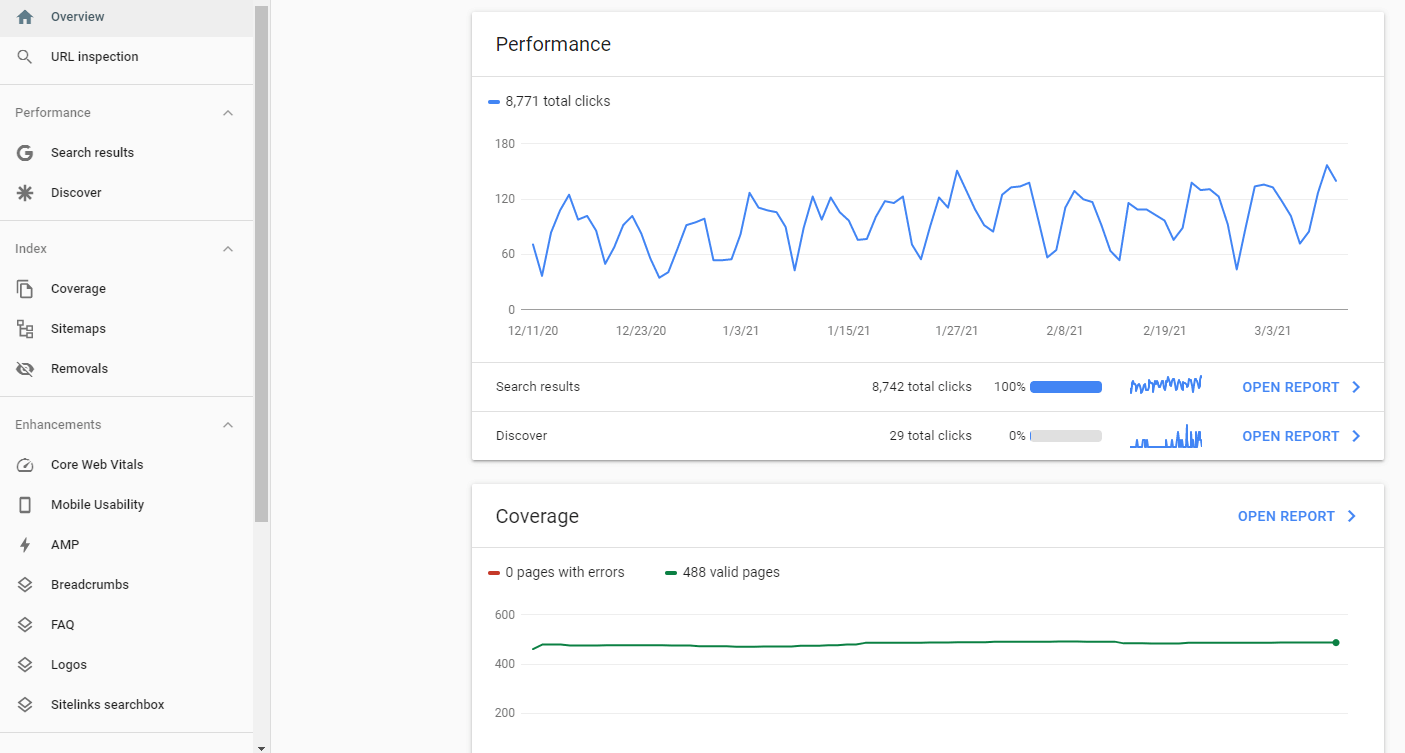This detailed performance graph, likely sourced from a Google tool, is displayed on a webpage with a clean white background. The layout includes a vertical navigation menu on the left, listing various sections such as Overview, URL Inspection, Performance, Search Results, Discover, Coverage, Sitemaps, Removals, Enhancements, Core Web Vitals, Mobile Usability, AMP, Breadcrumbs, FAQ, Logos, and Sitelinks Search Box. Small icons accompany each menu item, with certain sections like Performance, Search Results, and Enhancements featuring drop-down menus for additional options.

The main section on the right prominently displays the "Performance" report. At the top, it shows that the website has accumulated a total of 8,771 clicks. A bar graph beneath this summary spans from December 11, 2020, to March 3, 2021, featuring a fluctuating blue line to represent the varying number of daily clicks.

Further below, the report breaks down these clicks into different categories. "Search Results" account for 8,742 clicks, making up 100% of the total, while "Discover" contributes a smaller portion with 29 clicks, amounting to 0%. Additionally, a "Coverage" section highlights that the site has 488 valid pages, indicated by a steady green line. Buttons labeled "Open Report" in blue are available for more detailed information on Search Results, Discover, and Coverage.